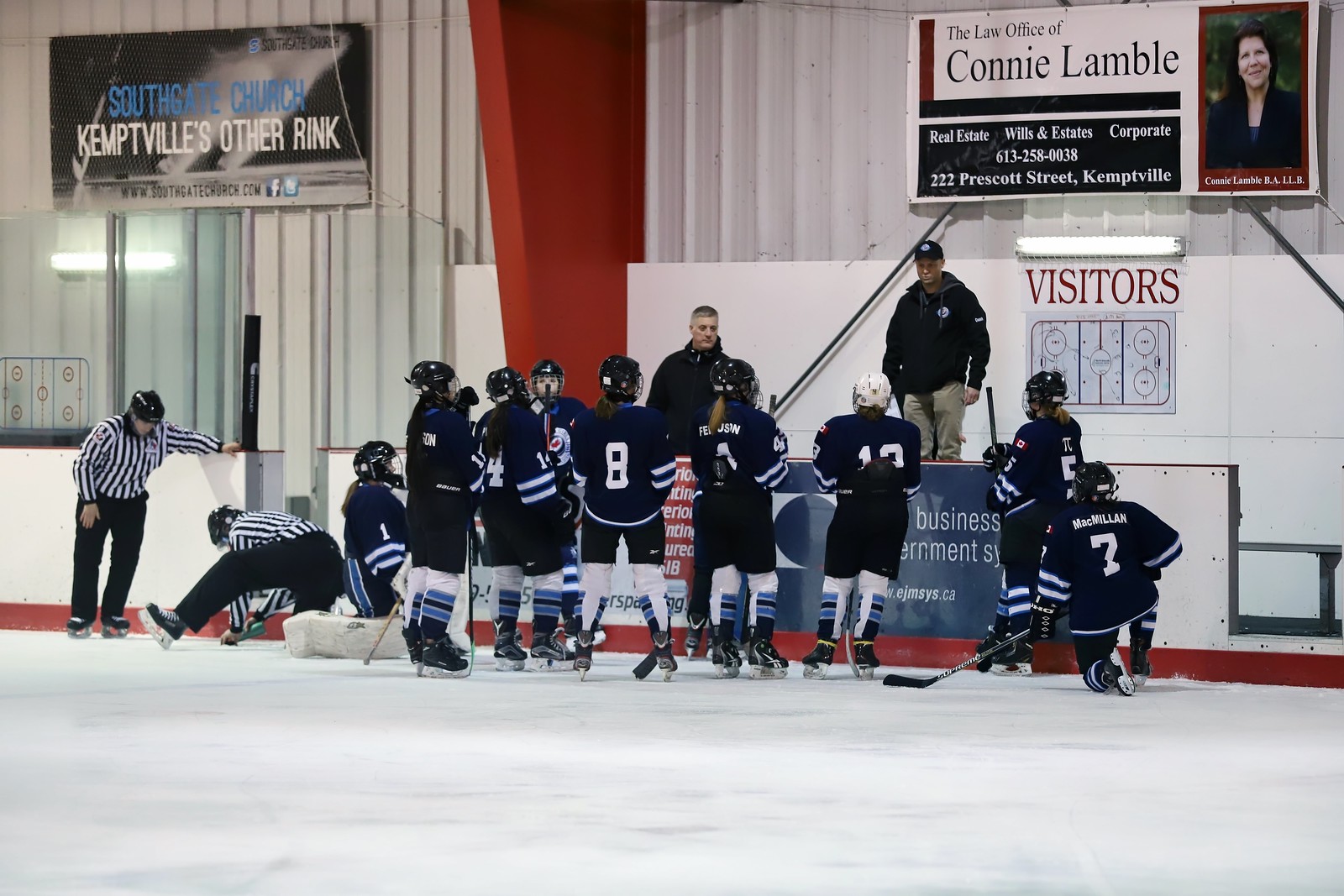This detailed image showcases a girls' ice hockey team, identifiable by their long hair, positioned on the ice in an indoor rink. They are dressed in blue uniforms, some with white names and numbers on the back, and equipped with their hockey sticks and skates. The team appears to be receiving a motivational speech from two coaches who are standing behind them on a platform, as hockey coaches typically do not go on the ice. The backdrop includes a "Visitors" light display in red, suggesting they are the visiting team, alongside an underneath board likely used for strategizing with markers. Advertisements line the walls of the rink, notably including one for the Law Office of Connie Lambeau, a real estate and corporate lawyer, and another for Southgate Church. The white-walled arena also features a few banners and two referees to the left - one stretching and the other attending to something on the ice, hinting at pre-game preparations. Overall, the photograph captures a vibrant moment of readiness and anticipation before the start of the game.